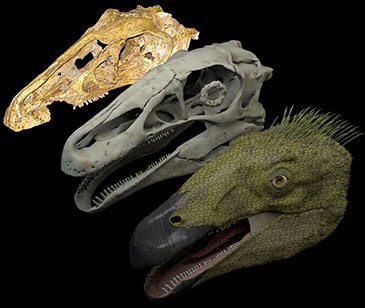The image showcases three dinosaur heads, each depicting different phases of reconstruction against a solid black background, arranged diagonally from top left to bottom right. The top-left head is a skeletal form rendered in a brownish-tan hue, with an elongated beak and a row of thin, small white teeth, lacking a lower jaw. In the middle, the head is more filled out, crafted from gray clay, replicating the skeletal structure but with additional mass to suggest musculature and other tissues. The bottom head is the most detailed and lifelike, featuring green scales, a black beak, small white teeth in an open mouth, and spikes resembling sprouting grass on its head, indicating a plausible appearance of the dinosaur when it was alive. All heads are oriented to the left, providing a comprehensive visual progression from fossil to fully reconstructed creature.